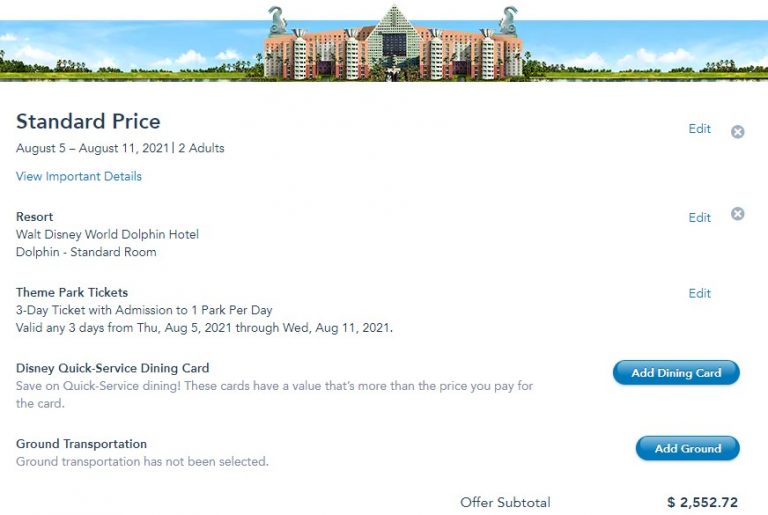The image showcases an order screen from a website. At the top, there's a banner displaying a vivid blue sky with green grass and foliage on the sides, framing a large, orange-colored building accented with white details. Below the banner, the details for the order are listed.

The first section reads: "Standard Price, August 5th through August 11th, 2021, two adults," followed by "View Important Details" and buttons for "Edit" and "Exit" on the right-hand side.

The next line features accommodation details: "Resort: Walt Disney World Dolphin Hotel, Dolphin Standard Room," with options to "Edit" and "Close" on the right. 

Following this, the theme park ticket information is provided: "Theme Park Tickets: Three-day ticket with admission to one park per day, valid any three days from Thursday, August 5th to Wednesday, August 11th," with an "Edit" button.

Further down, dining options are highlighted: "Disney Quick Service Dining Card: Save on quick service dining, these cards have a value that's more than the price you pay for the card," along with an "Add Dining Card" button.

Lastly, the ground transportation information indicates: "Ground Transportation: Ground transportation has not been selected," followed by an "Add Ground" button.

At the bottom of the screen, the order subtotal is displayed, amounting to $2,552.72.